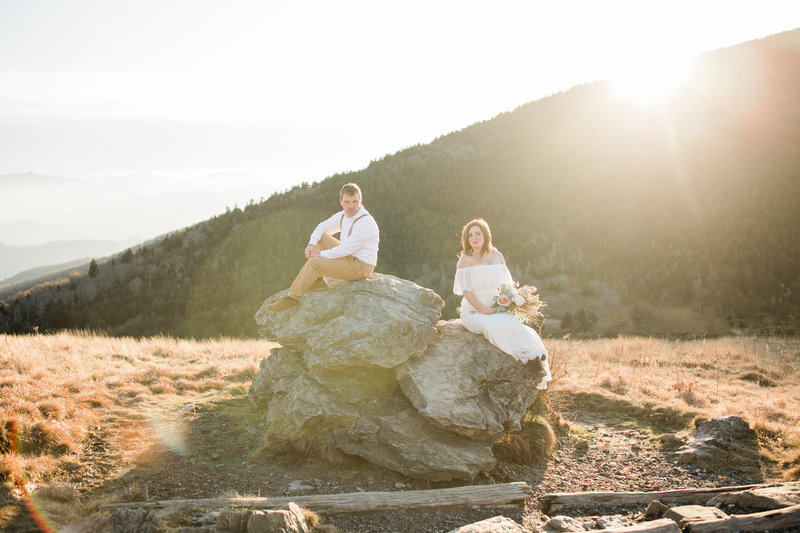This enchanting wedding photograph captures a couple in a serene, mountainous desert landscape. The scene is set against the backdrop of a large hill adorned with a mix of desert vegetation and a scattering of trees, all bathed in the golden hues of a setting sun. The couple is seated atop a collection of rugged rocks; the man sits slightly higher than the woman, creating a subtle yet charming composition. 

The woman, with her light brown hair gently framing her face, wears a shoulderless, short-sleeved white wedding dress. Resting a bouquet of flowers on her knees, she gazes softly at the camera. She is seated on the lower right rock, her legs casually positioned with her right knee slightly raised, revealing her brown shoes beneath the flowing dress.

The man, positioned on the left, sports a white dress shirt paired with tan pants, brown suspenders, and brown shoes. Sitting with one knee raised and his right arm resting on it, he looks directly at the camera with a relaxed demeanor.

Surrounding them is a quintessentially desert landscape — dry grasses and shrubs scattered around, capturing the essence of an Arizona-like biome. The setting sun behind the distant hill lends a natural lens flare to the photograph, enhancing its warm, romantic atmosphere.